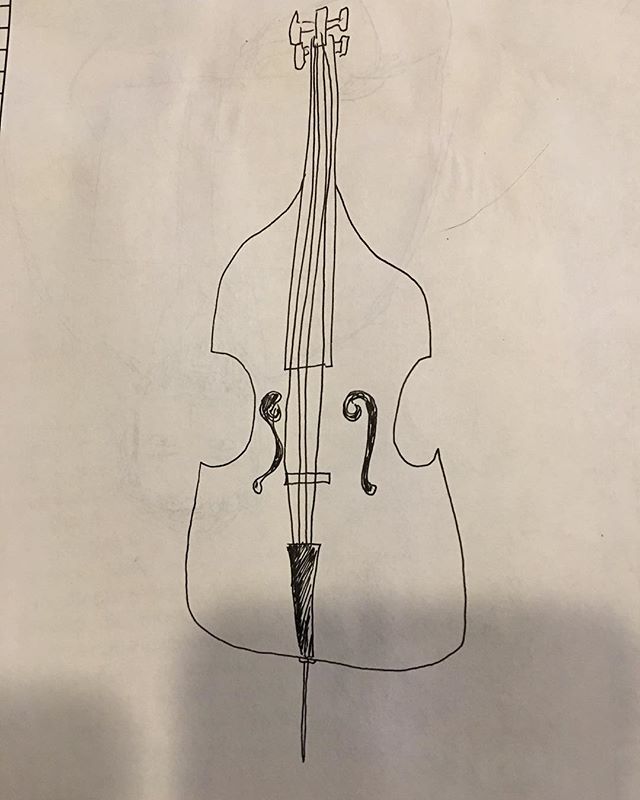A beautifully simplistic and elegant pen sketch of a cello graces the white background of this image. The artist has meticulously illustrated the instrument, capturing the essence of its form with remarkable clarity and precision. The cello is depicted with its signature features: the four taut strings stretching down the neck to the tuning pegs, the delicately crafted sound holes that open into its resonant chamber, and the single spike stand at its base. The contours of the instrument are evident with graceful indentations and hooks defining its sides, reflecting the classic silhouette of the cello. Additional sketches appear faintly on the left side of the paper, hinting at the artist's broader exploration of musical themes. A subtle crease in the paper adds to the charm, suggesting the artist's hands-on process. This minimalist yet thoughtful sketch offers a window into the artist's conceptual interpretation of the beloved stringed instrument.